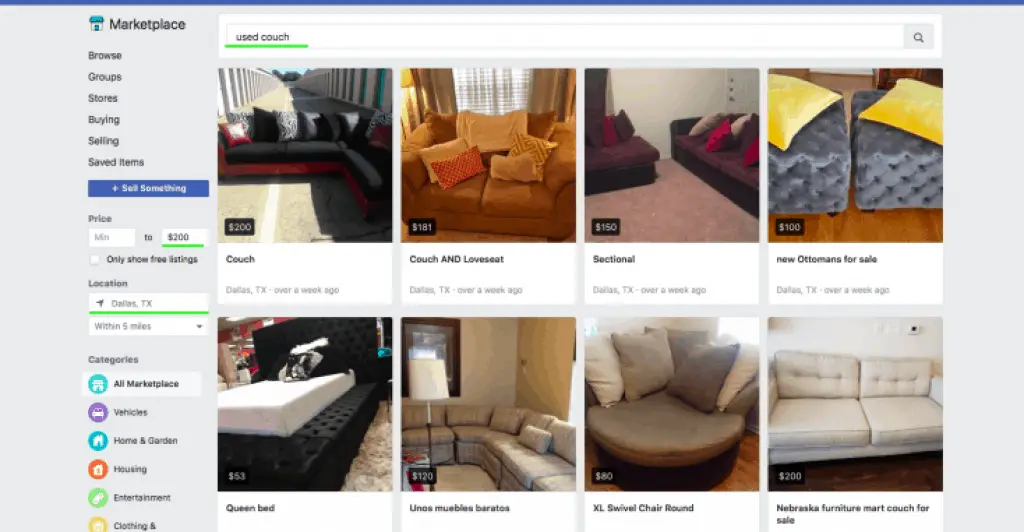This is a detailed screenshot of Facebook Marketplace. On the left-hand side, there is a navigation bar labeled "Marketplace." Available options include Browse, Groups, Stores, Buying, Selling, Saved Items, and a prominent blue button labeled "Sell Something." The search filters show a maximum price of $200 and the location is set to Dallas, Texas, with a drop-down menu to adjust the search radius.

The categories listed are All of Marketplace, Vehicles, Home and Garden, Housing, Entertainment, and Clothing, though the list is cut off and the final category is not visible.

On the right side of the screen is the search bar, currently focused on "used couch." Below the search bar, eight listings are displayed. The first row features a red and black sectional, a couch and loveseat sectional, and a new ottoman. The second row includes a queen bed, another sectional, an extra-large swivel chair, and a couch from Nebraska Furniture Mart.